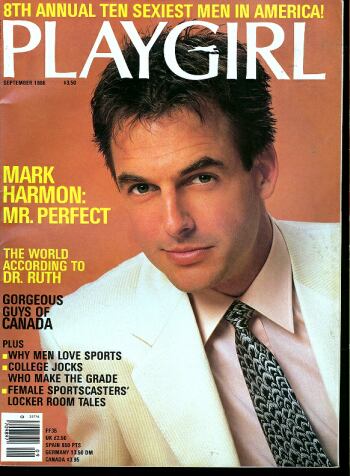This is an image of a magazine cover from Playgirl. At the top of the cover, the magazine's title "Playgirl" is prominently displayed in white font. Above the title, the feature "Eighth Annual Ten Sexiest Men in America" is highlighted in bold yellow print. The centerpiece of the cover is a photograph of Mark Harmon, with accompanying text describing him as "Mr. Mark Harmon, Mr. Perfect," rendered in yellow against a flesh-colored background. Harmon is pictured wearing a white coat, a pink shirt, and a black and white printed tie.

Beneath the "Mr. Perfect" caption, additional headlines are displayed, including "The World According to Dr. Ruth" in yellow letters on the same flesh-colored background. Further down, in bold black text, are the features "Gorgeous Guys of Canada" and an array of intriguing article titles such as "Why Men Love Sports," "College Jocks Who Make the Grade," "Female Sportscasters," and "Locker Room Tales."

In the lower-left corner of the magazine cover, there is a QR code for easy access to more content. This Playgirl issue notably features the Eighth Annual Ten Sexiest Men in America.